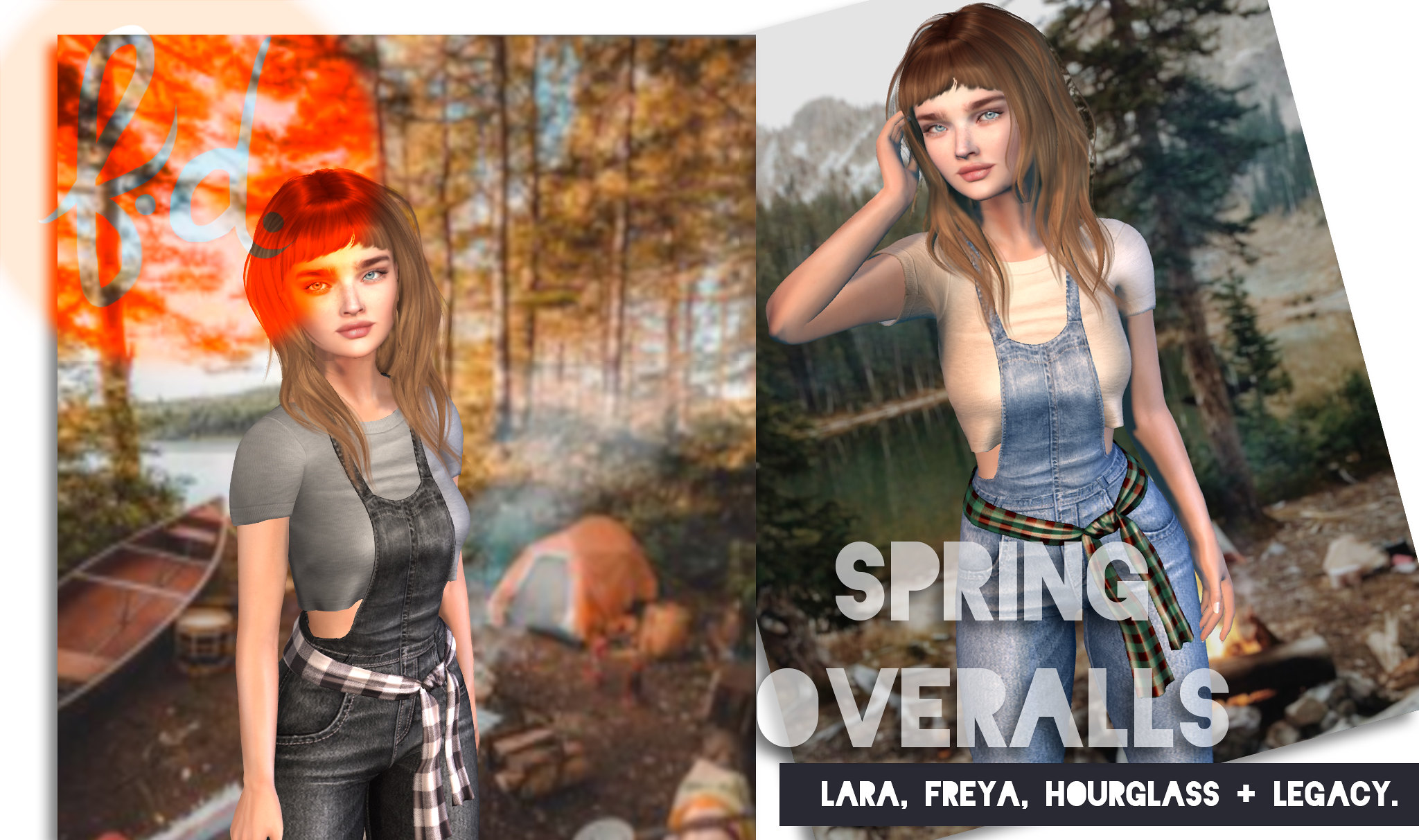This detailed computer-generated advertisement features two side-by-side animated images of the same young woman, set in picturesque outdoor scenes. 

In the left frame, she is depicted with long, brown wavy hair that falls past her shoulders, and she has bangs and blue eyes with a heart-shaped face. She wears a cropped gray T-shirt paired with black denim overalls. A black and white flannel shirt is tied around her waist, resembling a buffalo check belt. The background showcases a camping scene with autumnal trees, a shimmering lake, an orange tent, a canoe, and stacked firewood. An orange text overlay is partially visible in the upper left corner.

In the right frame, the same woman appears with her hand raised toward her ears, clad in a tan cropped T-shirt and blue denim overalls. Around her waist, she ties a green and brown check flannel shirt. The background reveals a serene lakeside scene reminiscent of Lake Tahoe, complete with evergreen groves, a calm lake, distant mountains, and a roaring campfire. Text on this image reads "spring overalls, Lara, Freya, hourglass, and legacy." 

The lush details and vibrant settings emphasize the advertisement’s focus on versatile, fashionable overalls suitable for camping and outdoor adventures.